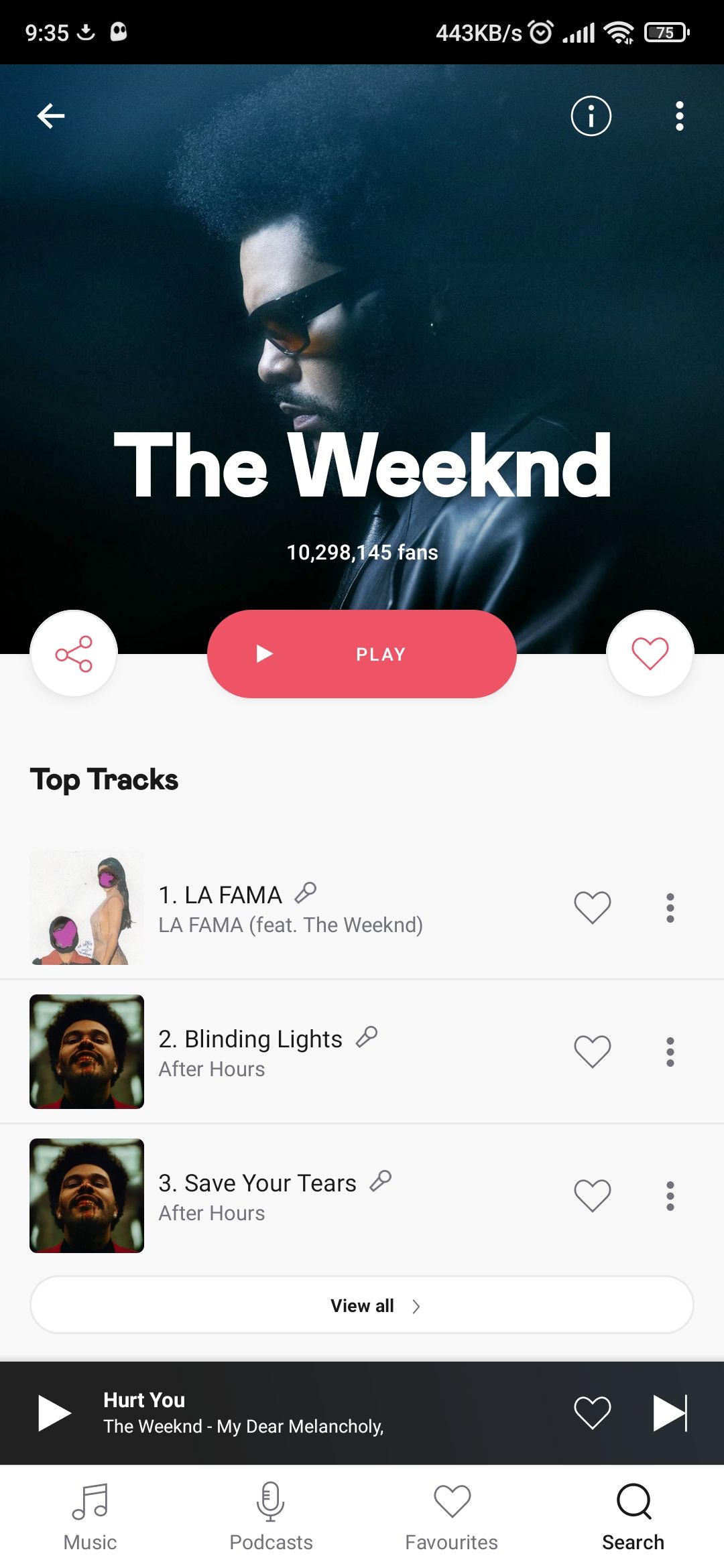This is a detailed caption for the described screenshot:

---

The screenshot, taken from a phone, prominently features The Weeknd, a well-known artist. The image showcases a black male artist with distinctive features: wearing sunglasses, sporting puffy Afro-like hair, and a goatee. He is turned sideways, revealing only the left side of his face. He appears to be wearing a jacket, possibly made of leather. 

In the upper left-hand corner of the screenshot, there's a back arrow pointing left. On the upper right-hand side, there is a circular icon with an exclamation point inside, followed by three vertical dots, representing additional options. Notably, there seems to be a visual effect resembling smoke near his hair.

Below the artist's image, there is a mention of his impressive fan count, which exceeds 10 million. A red, oval-shaped play button is present, along with a circular heart button and a share button on the left-hand side. 

Under these buttons, the text "Top Tracks" is displayed, listing three available tracks:
1. "La Fama" - accompanied by an image of two indistinct figures, possibly a drawing.
2. "Blinding Lights" - labeled under the album "After Hours", with its respective album art.
3. "Save Your Tears" - also with its corresponding image.

Additionally, there is a "View All" button and a play button specifically for the track "Hurt You."

---